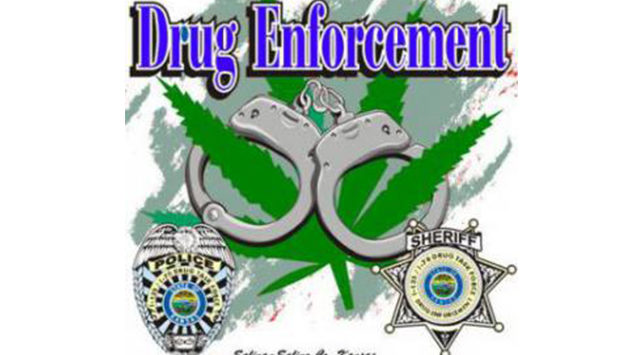The image appears to be an old, low-quality law enforcement poster aimed at combating drug use, specifically marijuana. At the top of the poster, the words "Drug Enforcement" are prominently displayed in a blue font outlined in white and yellow. Just below this text is a cartoonish depiction of a green marijuana leaf, which has silver or gray handcuffs around two of its leaves, symbolizing the crackdown on marijuana. In the bottom left corner is a police badge featuring an eagle, and in the bottom right corner is a sheriff’s star-shaped badge. The poster's background is primarily white with a smudged gray paint design, reminiscent of a 90s motif. The image also contains some illegible text at the very bottom.